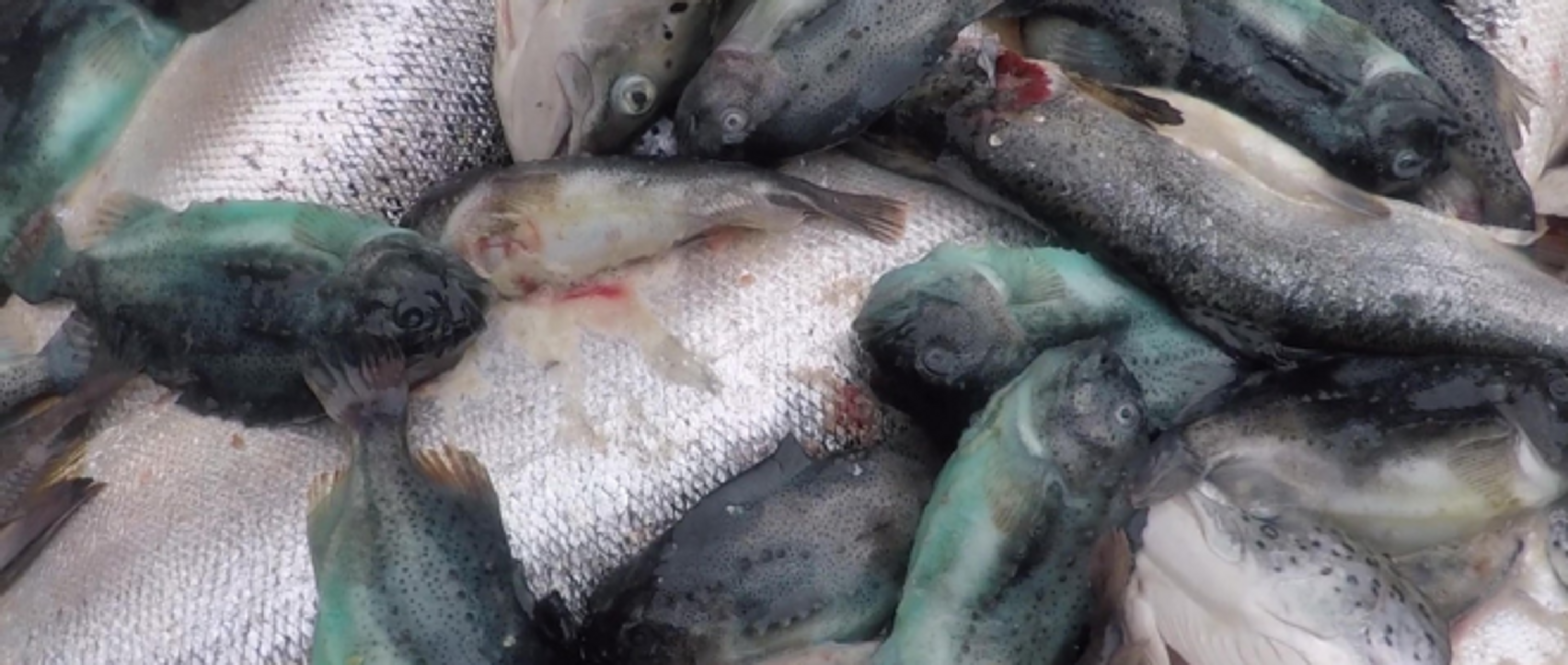This photograph features a chaotic pile of approximately ten dead fish, dominated by large silver-scaled specimens lying across the frame in a horizontal layout, obscuring any background surface. The central focus is on two large fish, likely tuna, with gray scales and white bellies, stretching from the bottom left to the top right of the image. Scattered atop them are smaller fish, including around six green and black fish with a distinctive jelly-like slime covering, clustered on the left-hand side and bottom of the frame. Interspersed among these are four or five white and gray fish, some speckled with blood likely from fishing hooks. The scene grimly highlights the textural contrasts between the slick, slimy surfaces of the green fish and the scaly, blood-speckled bodies of the larger ones, emphasizing the sheer mass and lifelessness of the catch.